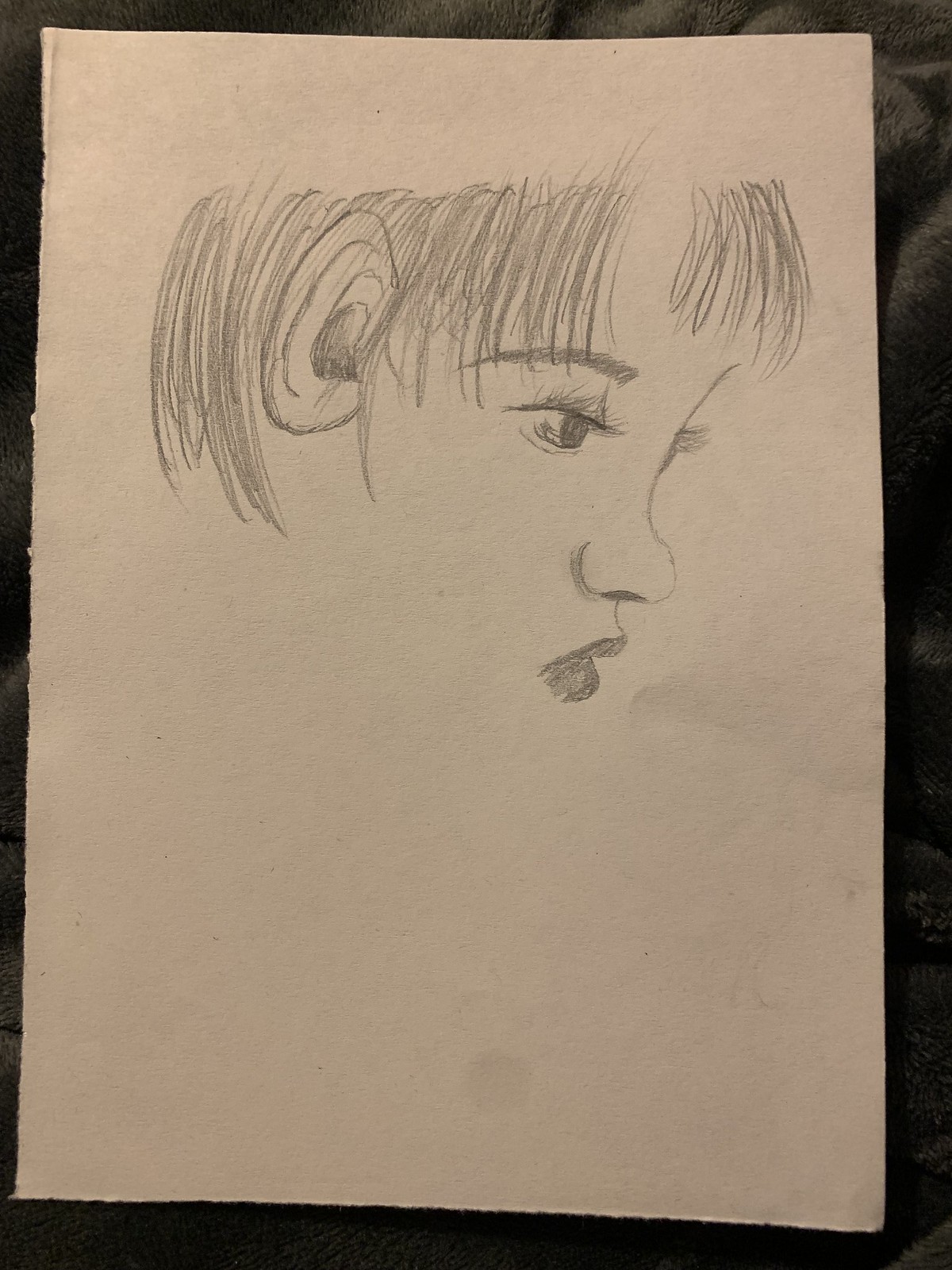Resting on a plush blanket, this image captures the beginning stages of a detailed pencil drawing on a piece of dark greyish-white construction paper. The drawing, done in shades of black and silver pencil, portrays a partial portrait of a female figure. The focal point is her forehead, adorned with meticulously drawn bangs that cascade down slightly past her ears. The drawing omits the top portion of her head, starting just around the forehead area.

One eye is particularly well-defined with a prominent eyebrow line, adding depth to the expression. Her medium-sized ears feature notable dark shading in the middle, creating a sense of realism. The nose is of moderate size, with subtle shadowing where it connects to the face, enhancing the three-dimensional effect. Her lips, darker and more detailed, provide a focal contrast against the lighter paper. The drawing abruptly ends just below the lips, leaving the image intriguingly incomplete.